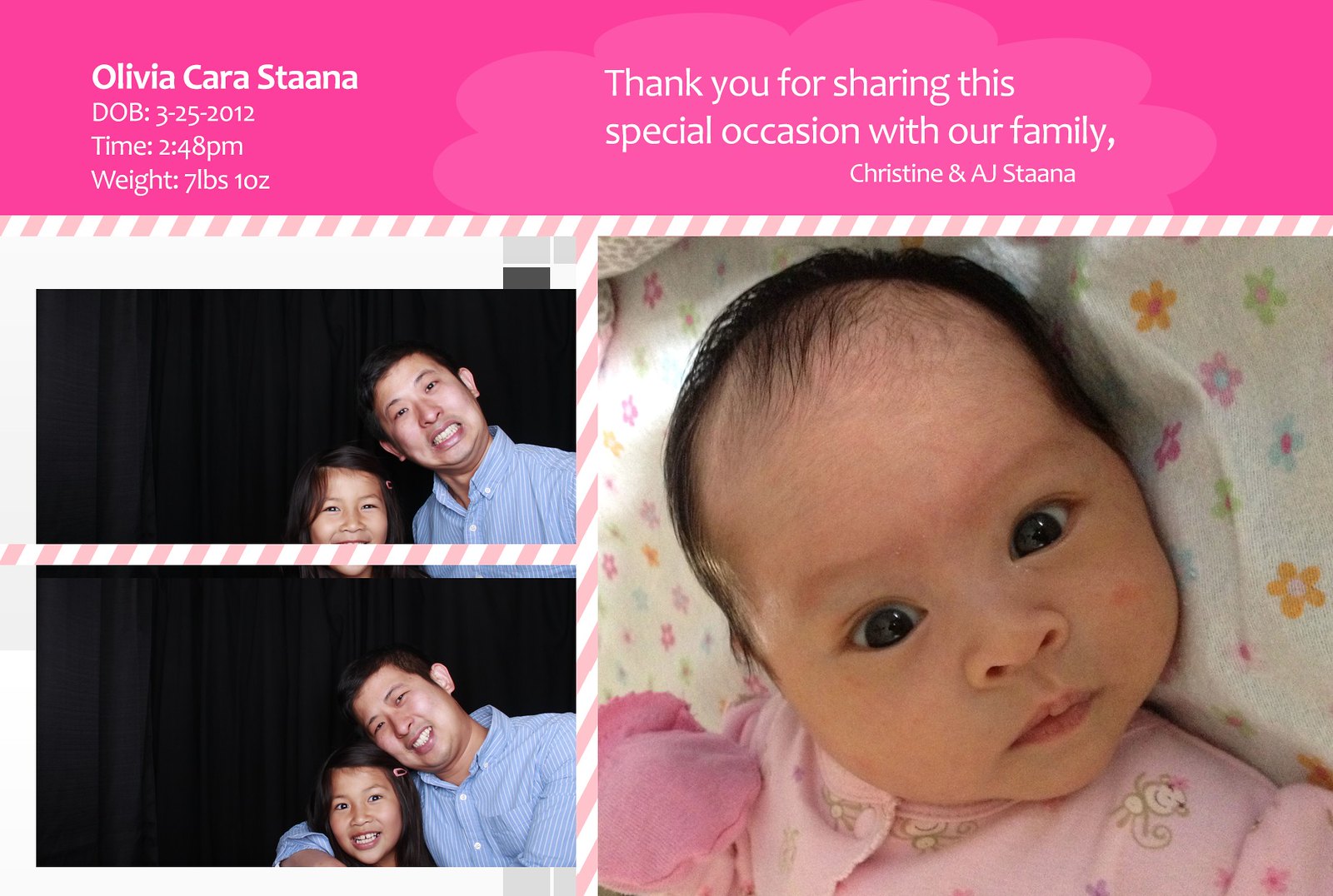This image appears to be a baby announcement card celebrating the birth of Olivia Cara Stana. On the top of the card, a pink bar features white text detailing her birth information: "Olivia Cara Stana, Date of Birth: 3-25-2012, Time: 2:48 p.m., Weight: 7 pounds 10 ounces." To the right of this text, a message reads, "Thank you for sharing this special occasion with our family, Christine and AJ Stana." The left side of the card includes two photos showing a man with a young girl, presented in different poses. On the right side, there's a picture of the baby, who has dark hair and dark eyes, looking straight into the camera. She is dressed in a pink sleeper outfit with her hands covered by something pink and lies on a white blanket adorned with colored flowers. The baby's onesie seems to have a monkey design. This horizontal card serves as a heartwarming welcome and announcement of Olivia's birth.